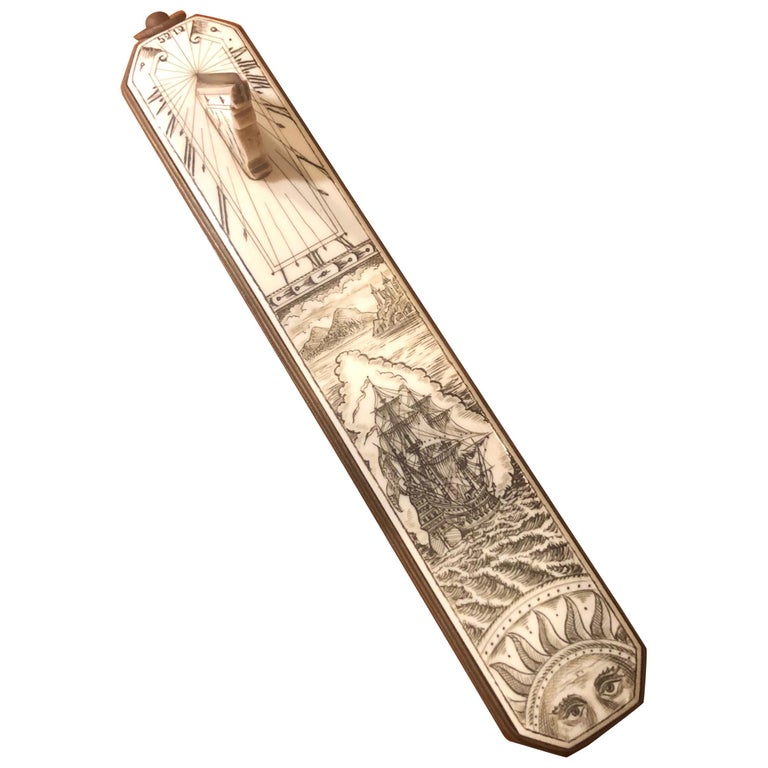The image showcases a photorealistic depiction of a narrow, tall tablet displaying classical artwork from the 15th or 16th century, resting lopsided to the left against a stark white background. The tablet, which has an ivory tone with brown and gray shadows, appears almost cylindrical and is detailed with various artistic engravings. At its top, there's an ivory knob, potentially part of a sundial mechanism, with numbers faintly visible. Below this, etched into the surface, is a depiction of a radiant sun with rays emanating outward. Further down, there's a detailed illustration of a ship braving rough waters, sailing away from islands adorned with castles or lighthouses. At the very bottom, partly visible, is a stylized sun with a face, adding to the intricate, historical feel of the piece. The entire tablet exhibits a harmonious blend of light, dark brown, and white hues.